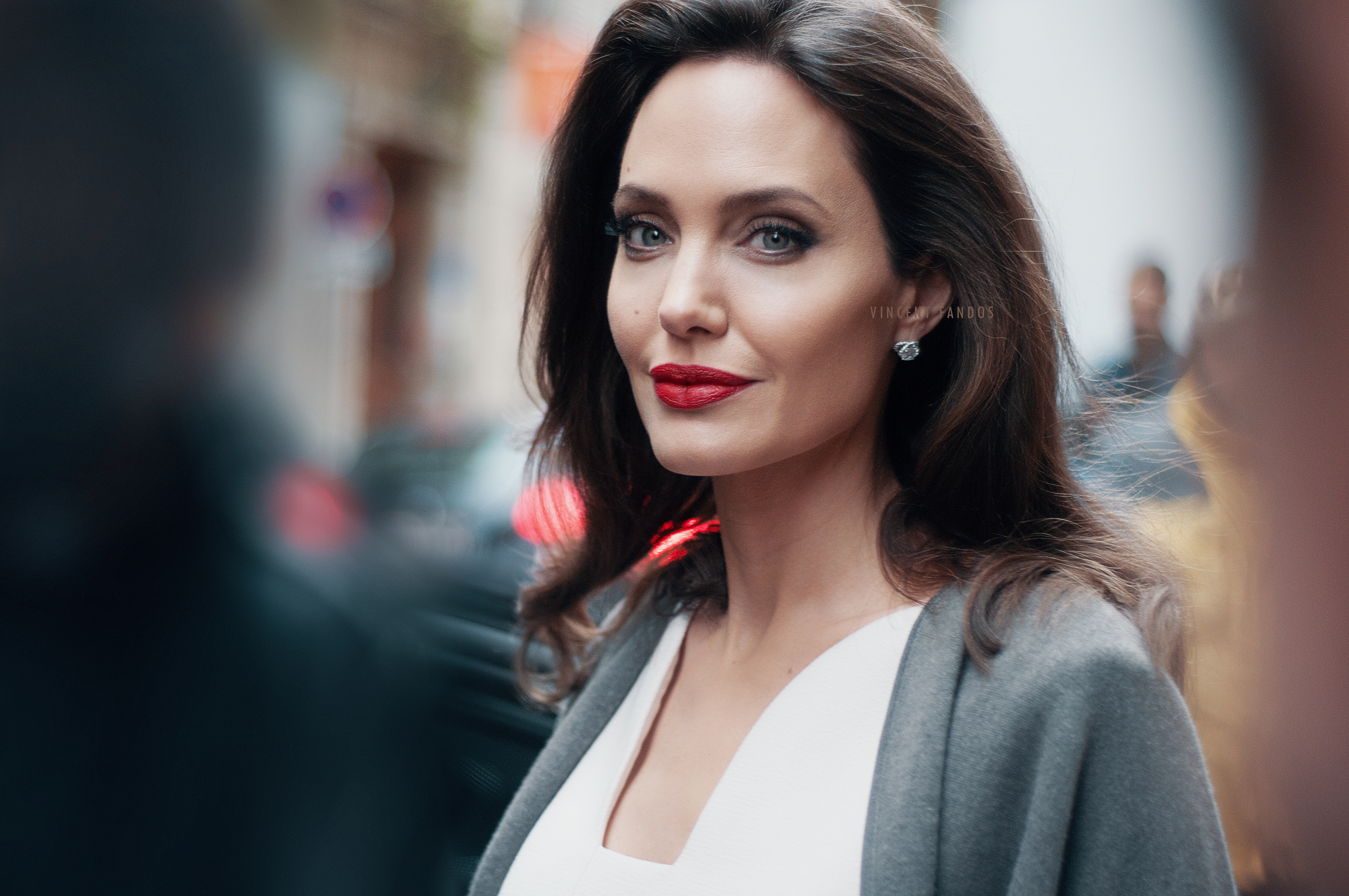The image captures a portrait of Angelina Jolie, centered prominently in the frame from her mid-chest upwards. She is looking directly at the camera, her chin and body subtly angled towards the seven o'clock position. Jolie, a middle-aged Caucasian woman, is easily recognizable with her signature blue eyes and red lipstick. Her voluminous, long brown hair cascades past her shoulders. She is dressed in a white shirt paired with a tan blazer. Notably, she wears a distinctive blue earring with a floral pattern. The background is artistically blurred, offering a hint of silhouettes, including what appears to be a person in a black coat or sweater on the left and some indistinct brown tones, suggesting an outdoor daytime setting. The overall image has a glamorous, almost hyper-realistic quality, accentuating Jolie’s features and attire.